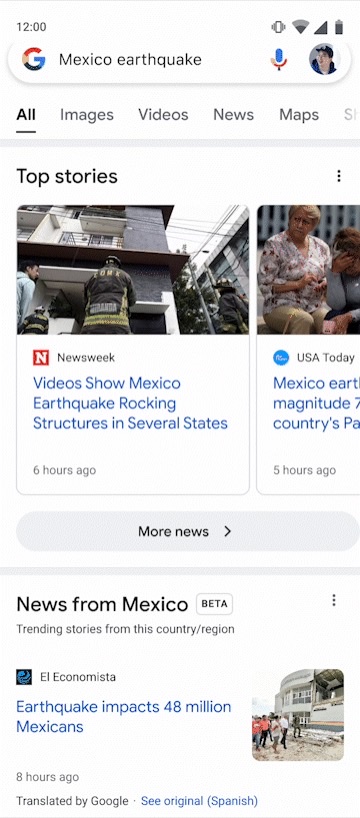The image depicts a news alert on a smartphone showing various updates and notifications. The phone displays the time as 12 o'clock, has a vibrating notification, full signal strength, almost full battery, but not a full WiFi connection. The main news headline concerns a recent earthquake in Mexico, with accompanying images and videos highlighting the aftermath. The visuals show rock constructions damaged in southern states, particularly Texas, around 6 hours ago. Additionally, there are reports of banditry in Mexico from 5 hours ago. The screen is populated with sections such as "images," "videos," "news," "maps," and "top stories." Among the visuals, soldiers are visible, and there are scenes of people standing amidst rubble, some wearing orange and white shirts, under a whitish sky. The overall theme of the notifications and images is the recent earthquake in Mexico and the ongoing situation, capturing the chaotic and distressed environment.